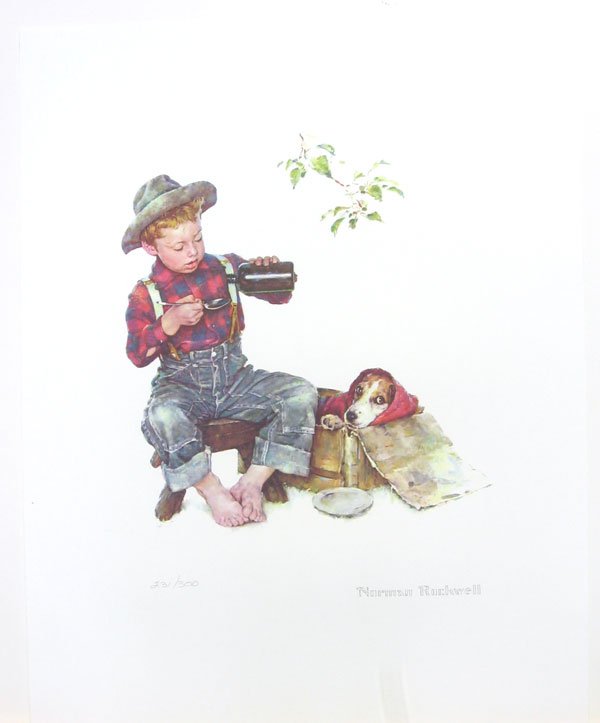This image is a Norman Rockwell illustration of a young boy and his beagle dog, featured on a book page with a white background and light gray border. The boy, who has short strawberry blonde hair and a brimmed hat, is sitting barefoot on a brown wooden stool. He is dressed in blue jean overalls with rolled-up bottoms, a red and blue plaid long-sleeve shirt, and suspenders with light-colored straps and dark brown attachments. The boy is looking down as he carefully pours a brown liquid from a glass bottle into a spoon held in his right hand.

To his right, inside a cardboard box, sits the beagle dog. The dog is adorned with a red bonnet that covers its ears and head, leaving its white snout and black nose visible. One of the dog's paws rests on the side of the box, and its expressive eyes gaze directly at the viewer. A white saucer is placed on the ground in front of the box. Above the boy and dog, a sprig of leaves hovers, creating a touch of natural detail in the scene. In the lower right corner, the artist's signature, "Norman Rockwell," appears in gray letters.